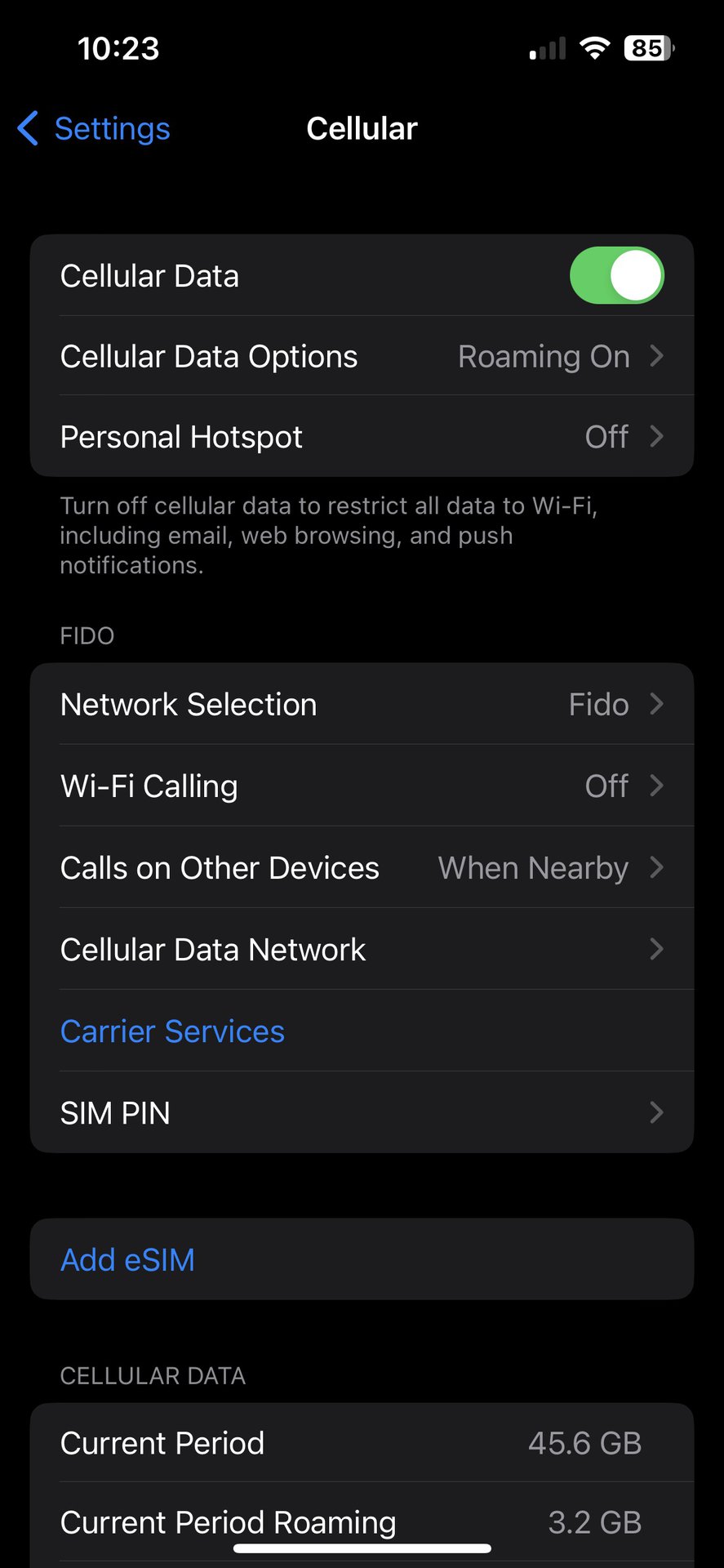The image displays a detailed screenshot of a cell phone's settings menu, focused on cellular settings. At the top of the screen, the time "10:23" is shown on the left, with status icons for cellular signal, Wi-Fi, and an 85% battery life on the right. Directly below is a blue "Settings" label flanked by a left arrow on a white background.

Centrally located in the image is the heading "Cellular" on a black background, indicating the active section. The first option listed is "Cellular Data," which is toggled on and highlighted in green. Following this, a series of settings are displayed, aligned to the left:

- "Cellular Data Options" with "Roaming On" and a right arrow.
- "Personal Hotspot" is listed as off, accompanied by a right arrow.

A descriptive note below informs users: "Turn off cellular data to restrict all data to Wi-Fi including email, web browsing, and push notifications."

Following this note, the carrier "FIDO" is specified in capital letters. The "Network Selection" option shows "FIDO" with a right arrow. Additional options include:

- "Wi-Fi Calling," which is off, with a right arrow.
- "Calls on Other Devices" is set to "When Nearby," with a right arrow.
- "Cellular Data Network" with a right arrow.
- "Carrier Services," highlighted in blue.
- "SIM PIN" with a right arrow.
- "Add eSIM," in blue.

Lastly, the data usage details are provided:
- "Cellular Data" section lists "Current Period" with 4.6 GB used.
- "Current Period Roaming" showing 3.2 GB used.

A darkened divider at the bottom of the screen marks the end of the visible settings.